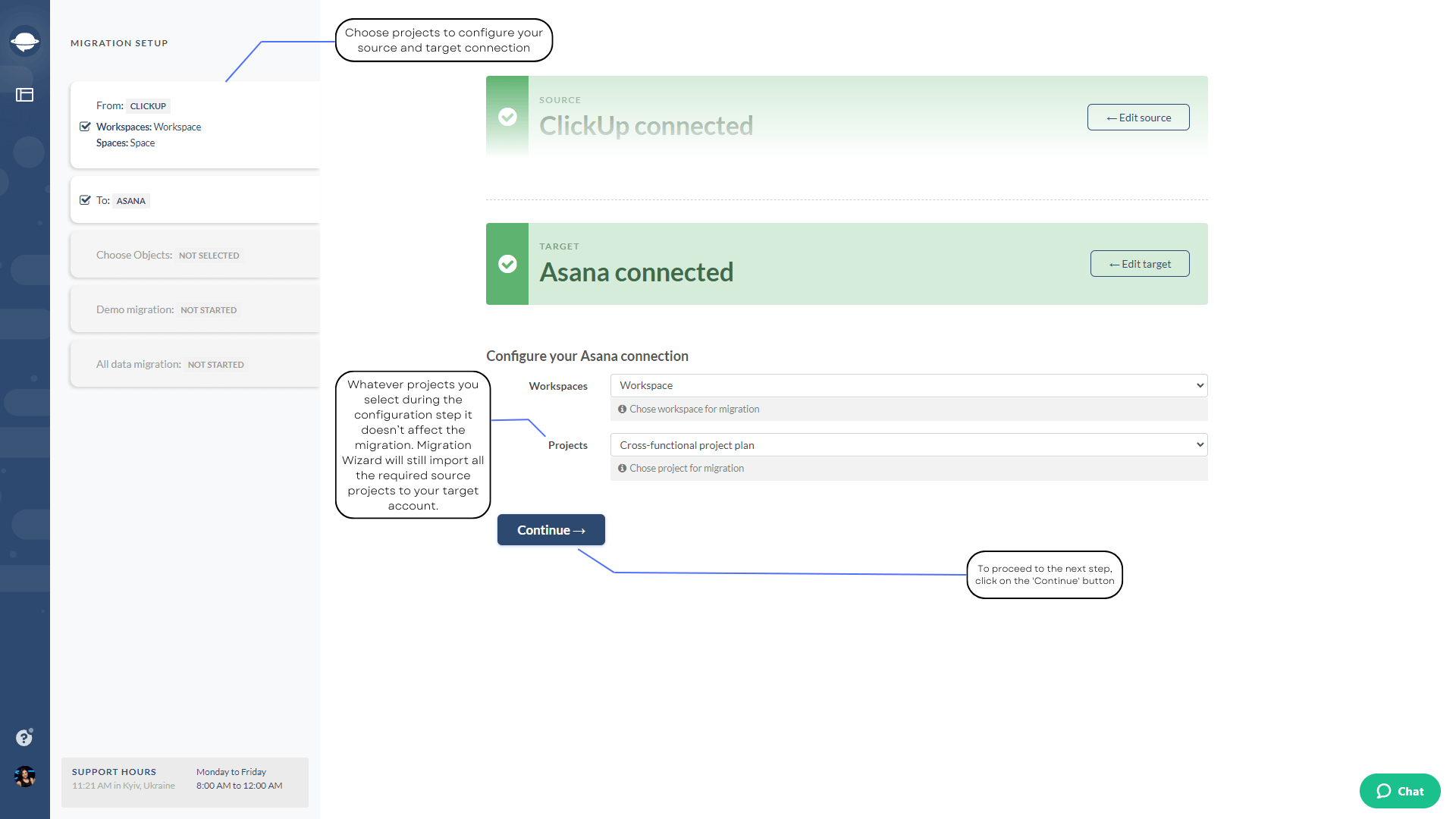This image appears to be a screenshot of a user interface, possibly from an app or website related to project management, most likely from ClickUp Workspaces. In the upper-left corner, there is faint and blurry text that reads "Migration Setup." The layout features a prominent blue column on the left side of the screen. At the bottom of this column, there's a circular avatar image of a woman, accompanied by a speech bubble with unreadable text.

Towards the center of the image, a prominent blue header contains partially legible text that starts with "Choose projects to configure your," followed by text that is difficult to discern. To the right, there are two green rectangles:

1. The first green rectangle reads "ClickUp Connected" with a white circle containing a green checkmark on its left side. Adjacent to this is a blue outlined rectangle labeled "Edit Source."
2. The second green rectangle reads "Asana Connected" with another white circle featuring a green checkmark on its left side. Below this, it instructs "Configure your Asana Connection" and features a blue rectangle below that reads "Continue."

A blue line extends downward from the "Continue" button, leading to a bubble with undiscernible text. Finally, at the very bottom of the interface, there is a small green circle labeled "Chat." 

The screenshot showcases a user navigating through a migration setup process involving ClickUp and Asana integrations._detailed remainder of the text.